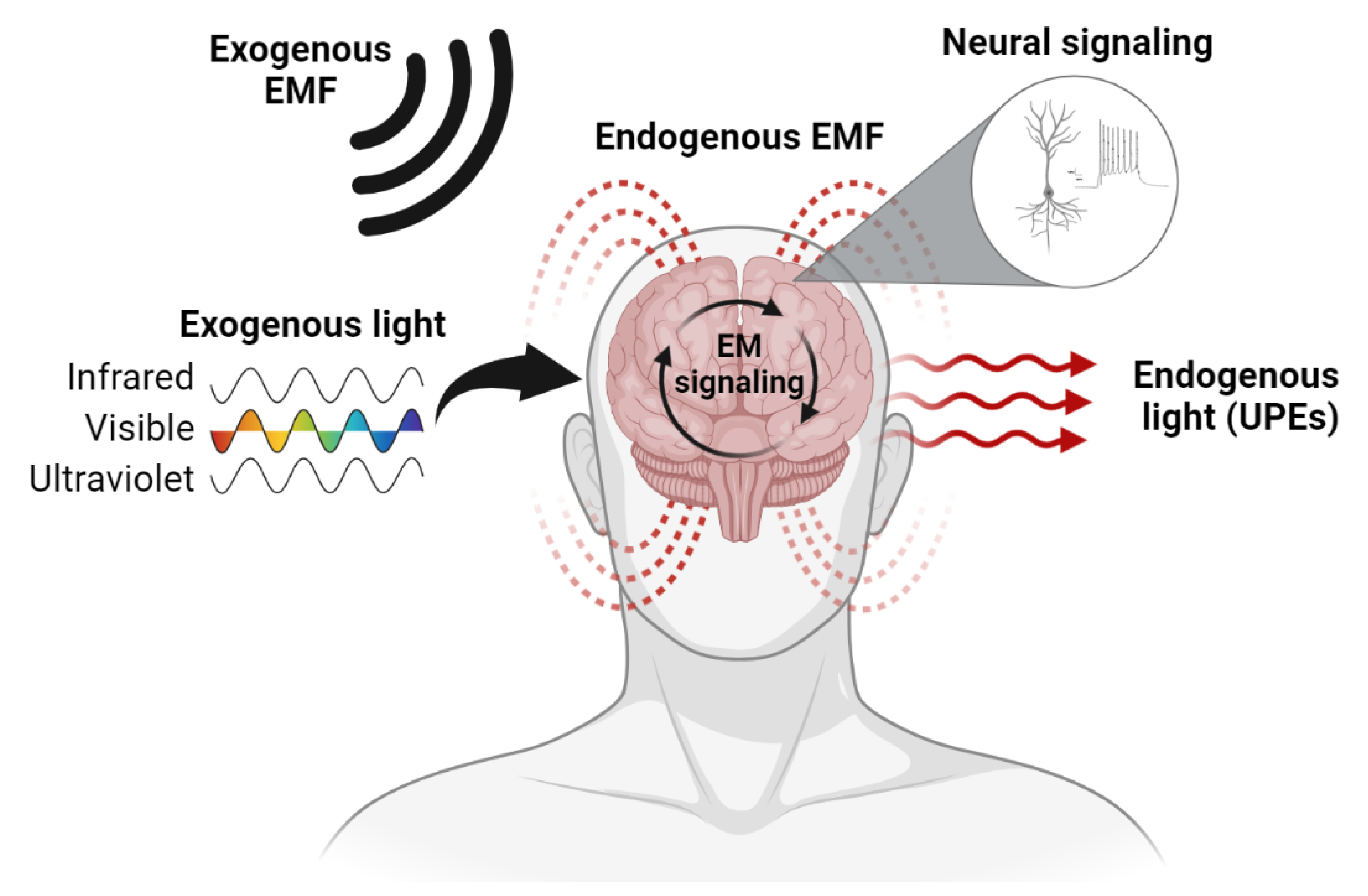This detailed illustration, set against a white background, appears to depict the complex interactions between the human brain and various types of electromagnetic (EM) signals and light frequencies. Central to the diagram is a featureless silhouette of a human figure, with a particular emphasis on the head and brain. The brain is highlighted in pink and features a circular, cyclical diagram labeled "EM Signaling."

Atop the brain section, the label "Endogenous EMF" can be seen. Surrounding the brain are various labels and arrows depicting different external and internal influences: "Exogenous EMF" and "Neural Signaling" to the right, and "Exogenous Light" (including subdivisions like Infrared, Visible (ROYGB color spectrum), and Ultraviolet) to the left. To the right of the brain, there's an indication of "Endogenous Light (UPES)."

Red, wiggling arrows emerge from the brain, signifying "Endogenous Light or UPEs." There are also detailed diagrams pointing to a magnified section depicting a neuron, annotated as "Neural Signaling." This comprehensive illustration generally conveys how external electromagnetic fields and light (exogenous) impact neural signaling within the brain and how this subsequently translates into internal (endogenous) electromagnetic frequencies and light.